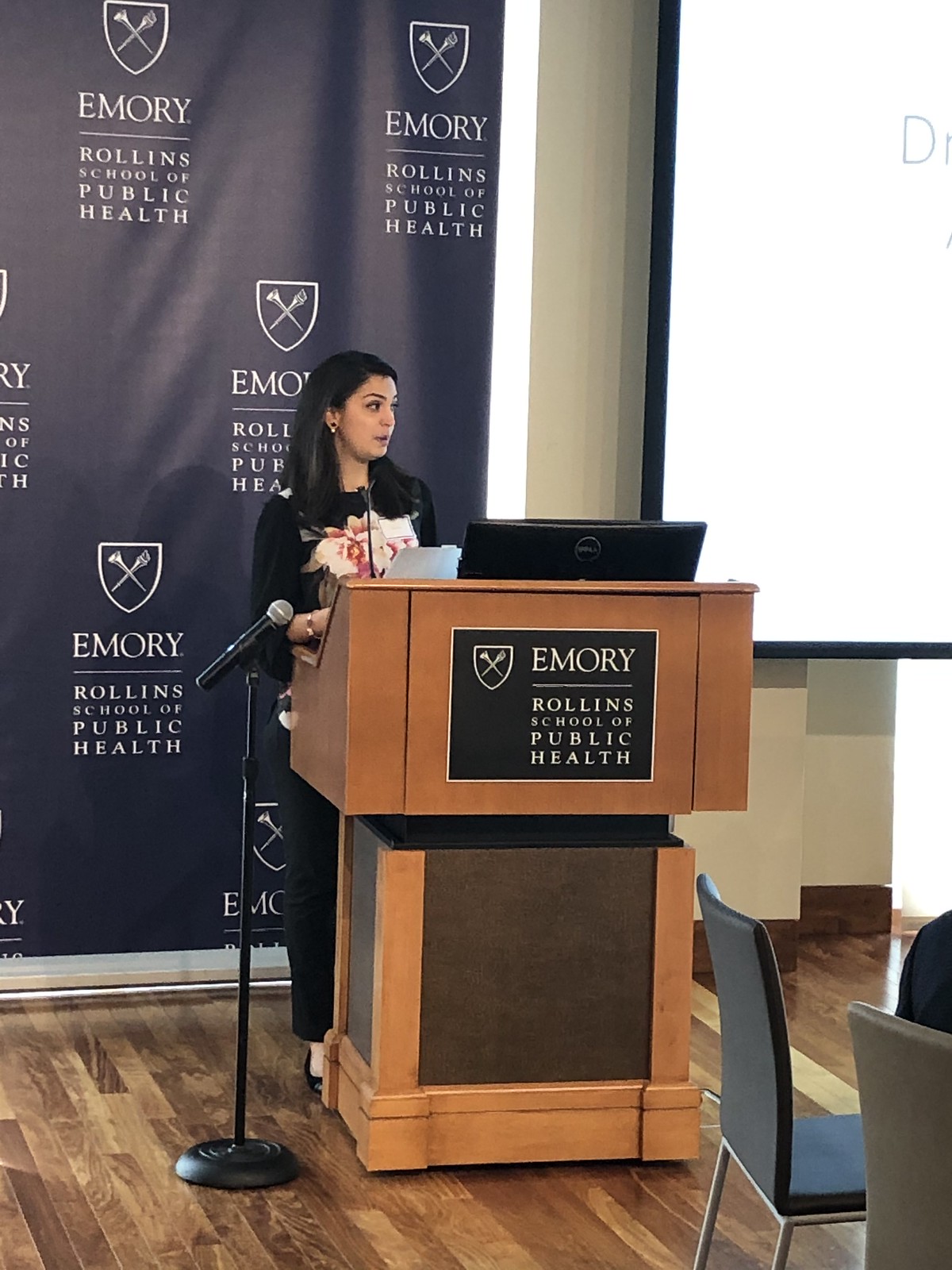In the image, a young woman, possibly in her 30s, stands behind a large, light brown wooden podium with a black microphone on its left side and a smaller microphone placed directly in front of her. She has long dark hair and is dressed in a black long-sleeve blouse adorned with a floral pattern, paired with black pants and black shoes. The podium bears the inscription "Emory Rollins School of Public Health" in white lettering, accompanied by a shield emblem featuring crossed torches. She has a laptop open on the podium, suggesting she is giving a lecture or presentation, potentially at a conference or educational event. Behind her, a blue banner reiterates the name "Emory Rollins School of Public Health" along with the emblem. To the right side of the podium, there is a projection screen with some partially visible text, and in front of the podium, there are a couple of black chairs. The floor is dark brown, enhancing the setting's professional atmosphere.